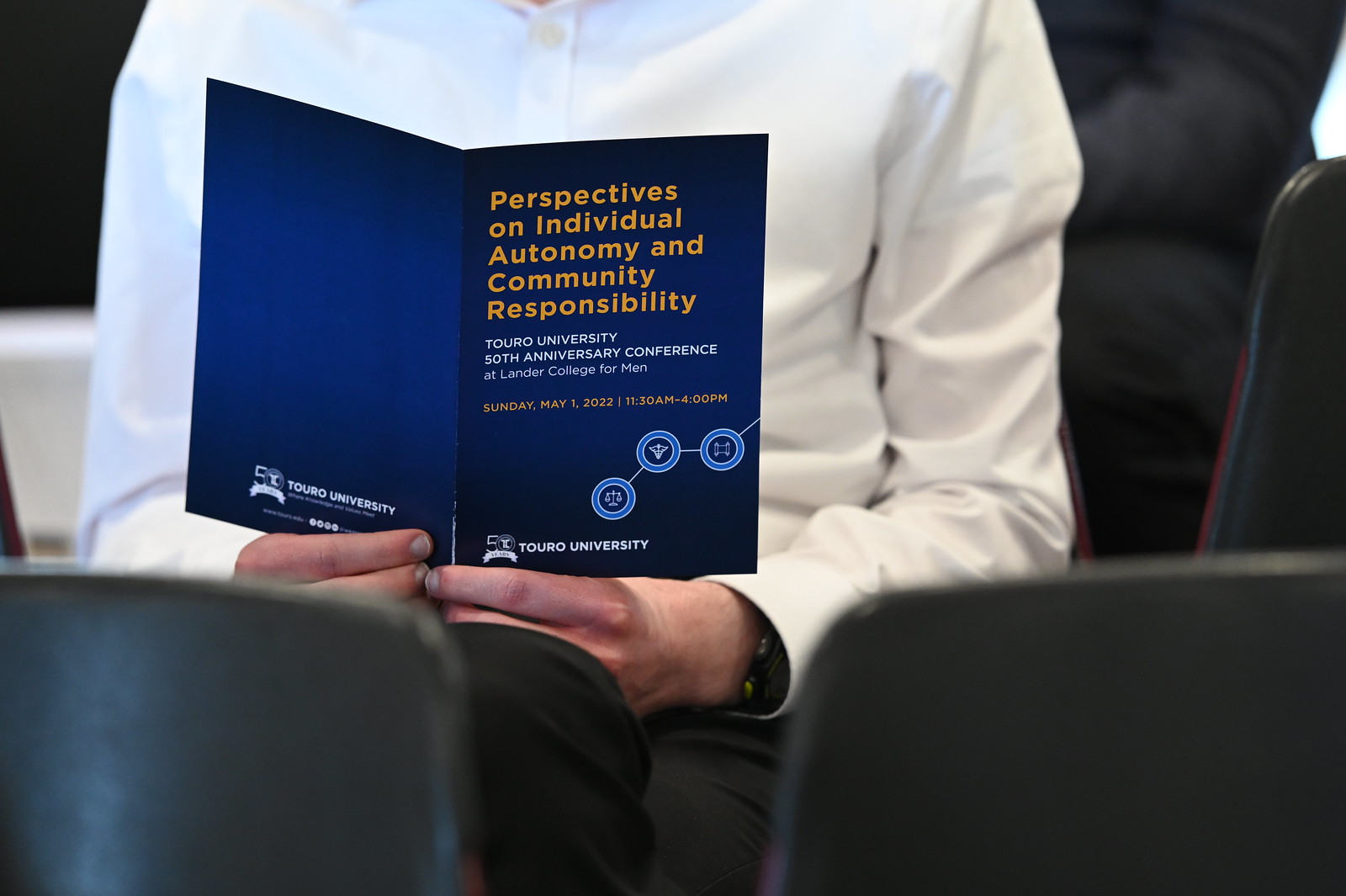This indoor photograph captures a close-up of a man seated in a chair, possibly in a waiting area or conference setting, reading a pamphlet. The image is focused on the man, who is wearing dark pants and a white dress shirt, with a watch visible on his wrist. The man is holding a blue fold-out flyer with both hands, which reads, in yellow text, "Perspectives on Individual Autonomy and Community Responsibility." Below this, in white text, it states, "Toro University 50th Anniversary Conference at Lander College for Men," followed by the date and time, "Sunday, May 1, 2022, from 11:30 a.m. to 4:00 p.m." The flyer also features various icons representing scales, medical symbols, and technology. The image is framed from the man's waist to his neck, obscuring his face. The foreground shows the blurry tops of two other chairs, and behind the man, faint outlines of more seating or possibly another person are visible.